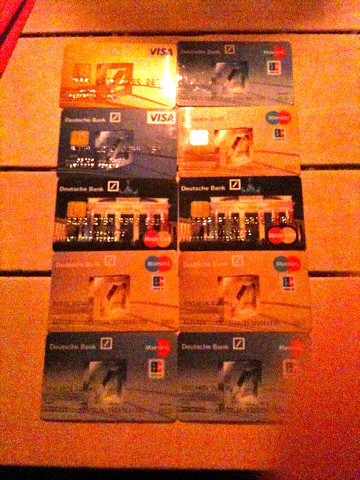The photo appears to be taken on a wooden platform, likely a picnic table, featuring distinct horizontal slats of a reddish-orange hue with black gaps between them. In the upper left corner, there is an additional red and black detail. The main focus is on ten credit cards arranged side-by-side in two rows of five. The cards include eight MasterCard and two Visa, differentiated by their colors and designs. Four of the cards are gold-colored, four are gray, and two are black. Most of the card designs feature indistinguishable images, possibly due to the poor quality and darkness of the photo, though one card clearly depicts a building with tall columns. The varied backgrounds and potential artistic elements suggest they are part of a collection showcasing different card designs.